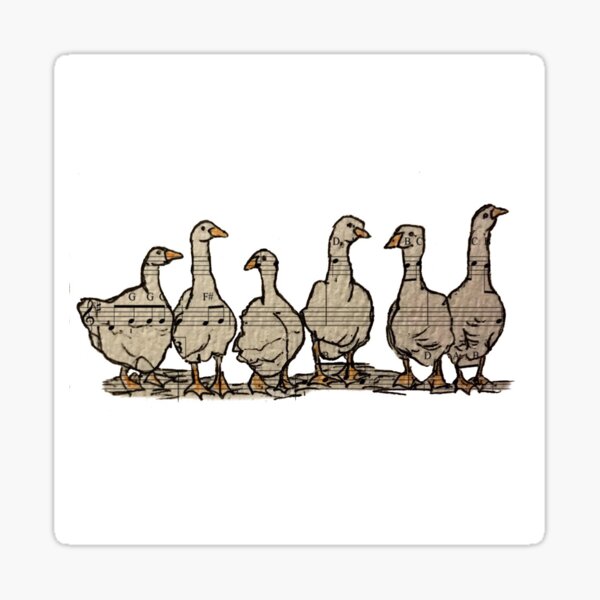This is a square image against a white background showcasing a drawing of six geese. The geese, standing on a slightly textured dirt ground, vary in height and are facing different directions—four to the right and two to the left. They all have gentle orange beaks and feet. Each goose is intricately decorated with sheet music, creating a unique pattern where the notes progress from one goose to the next, making it seem as if the sheet music was layered over their bodies and then cut out. The texture of the geese suggests a paper-like quality, and the artist has added shading around their legs to give depth. The overall composition of the geese, standing in adorable poses and seemingly poised for a performance, adds a charming and whimsical touch to the artwork.